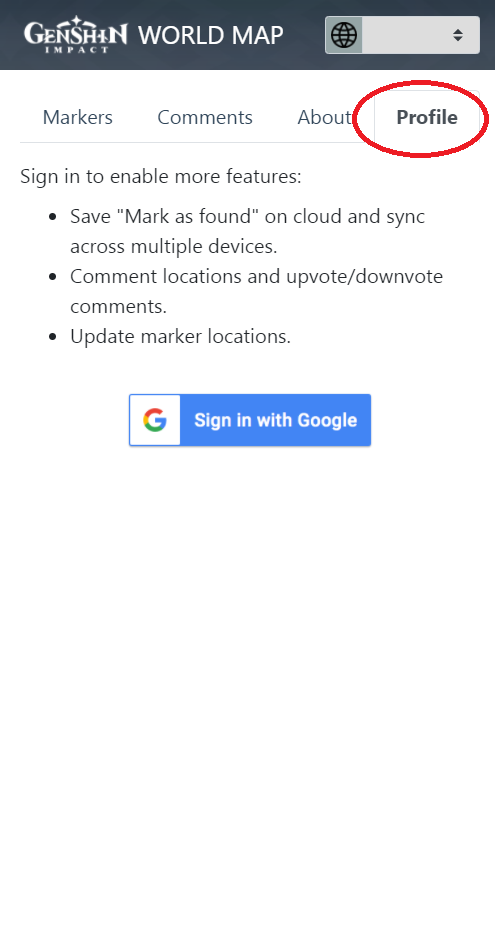The image features a user interface for a Genshin Impact world map tool. At the top, there is a black border displaying the title "GENSHIN IMPACT" in white letters. To the right, in larger white capital letters, it says "WORLD MAP." Adjacent to this, there's a gray square with a globe icon, followed by a white rectangular box featuring a drop-down menu button.

Below this, there are tabs labeled "MARKERS," "COMMENT," "ABOUT," and "PROFILE," with "PROFILE" in bold black letters circled in red. A light gray horizontal line separates this section from the area below.

Under the line, text prompts the user to "SIGN IN TO ENABLE MORE FEATURES:" followed by a list of bullet points. These are:
- "SAVE MARKERS FOUND ON CLOUD AND SYNC ACROSS MULTIPLE DEVICES"
- "COMMENT LOCATION AND UPVOTE/DOWNVOTE COMMENT"
- "UPDATE MARKER LOCATION"

At the bottom of the image, there's a white box with a blue rectangular button to its right. The button contains white text that says "SIGN IN WITH GOOGLE," and the box features a stylized "G" in the center.